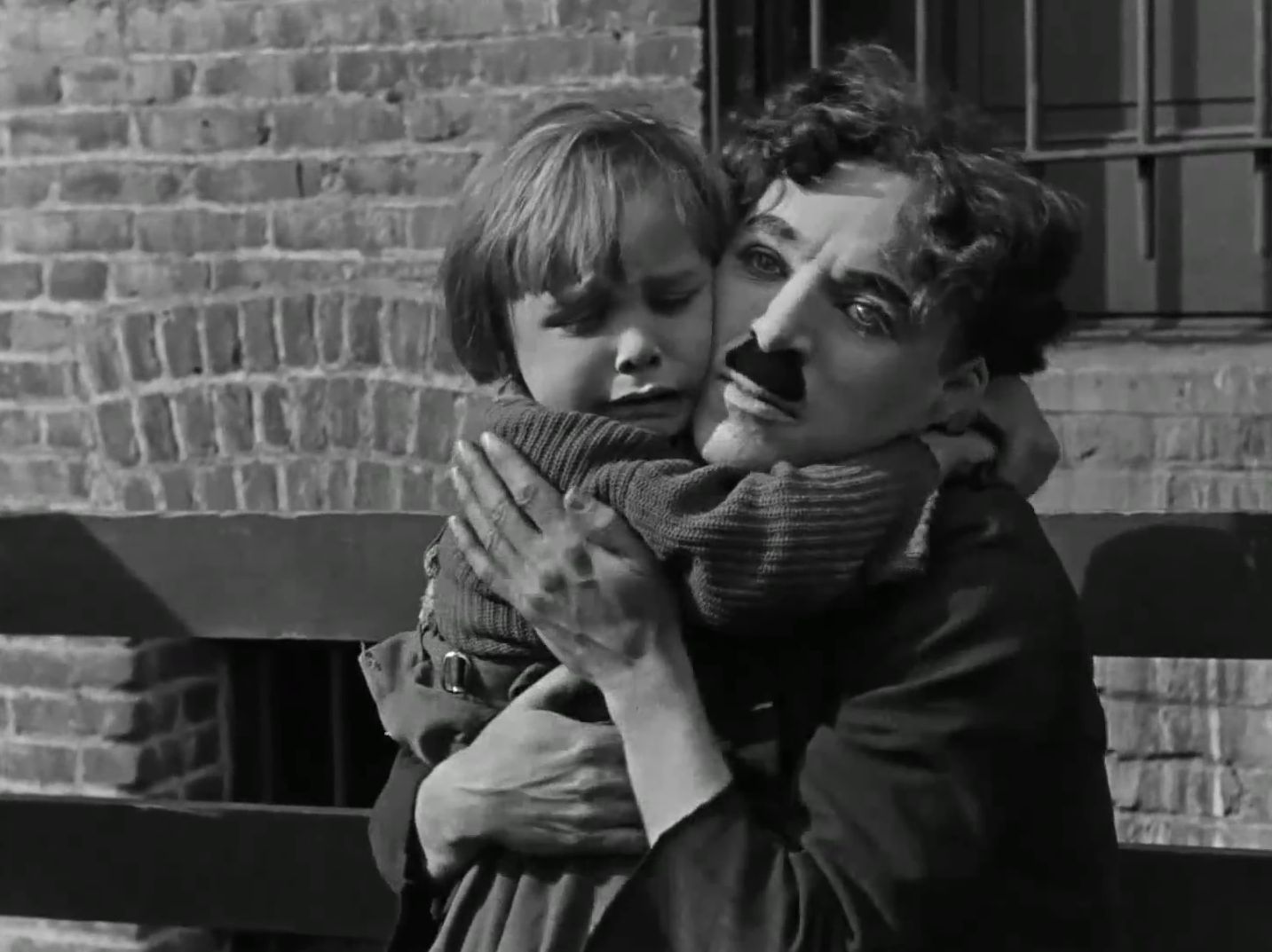In this evocative, high-contrast black and white photograph, the iconic early 20th century actor Charlie Chaplin is depicted holding a small child. Chaplin, identifiable by his distinctive thick mustache and curly dark hair, is dressed in his characteristic tramp attire, sans hat and cane. His expressive face appears somber, capturing the gravity of the moment. The child, with a pageboy haircut, is weeping, eyes closed, and clings to Chaplin, their faces touching in a heart-wrenching tableau. They are closely embraced, creating a poignant contrast between the hardened adult and the vulnerable child.

The backdrop of the photo is a dilapidated urban scene, with a brick building featuring prominently. Visible to the right is a window secured with iron bars, suggestive of a lower socioeconomic setting. Additional elements, such as wooden planks and another barred window in the lower left, further enhance this narrative of struggle and resilience. The daylight setting, possibly enhanced by studio lighting, bestows clarity and depth upon this expertly staged professional shot. From details such as their attire and the grayscale medium, the image appears rooted in the era spanning from the 1930s to the 1950s. The overall setting and careful framing lend the photograph a cinematic quality, likely a still from one of Chaplin’s films, capturing an intimate, emotional moment between the characters.